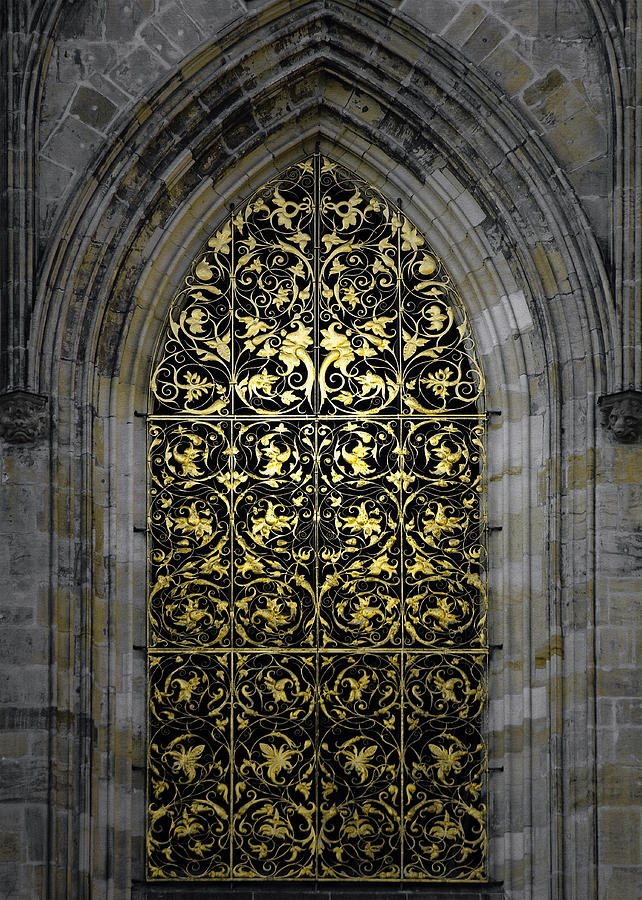This photograph captures a detailed view of a stained-glass window, likely located in a church. The window, set within an archway, features a pointed top and an intricate design dominated by dark maroon and gold colors. It is segmented into three sections: the top pointed section, a rectangular middle section, and another rectangular section at the bottom. Gold floral patterns, potentially representing flowers and plants, adorn the window without any discernible religious symbols. Horizontal bars traverse the window panes, and a gold-colored ledge is visible at the very bottom. This striking stained-glass window is framed by stonework that recedes backward toward the window area, complementing the overall design.